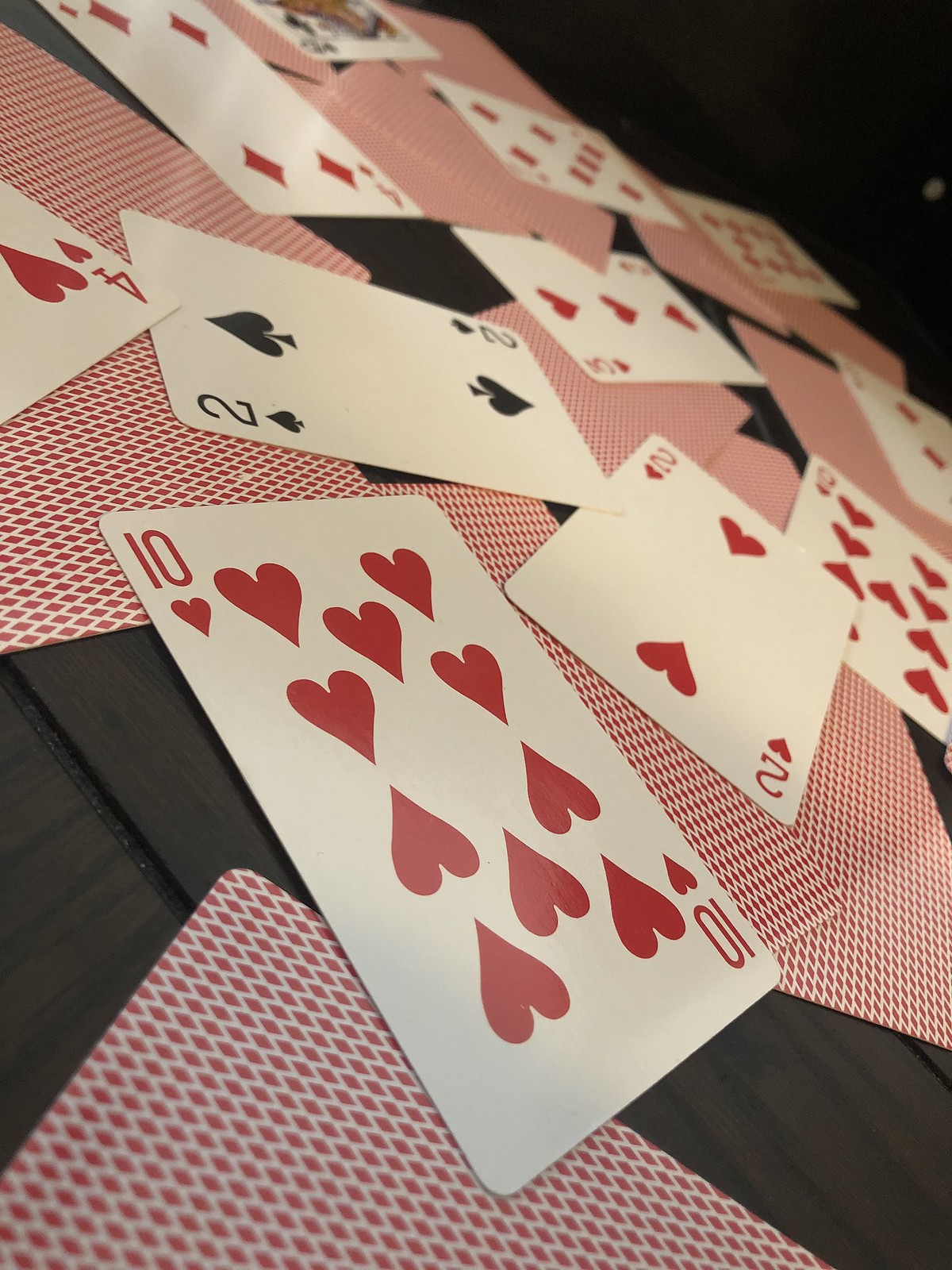In this image, a neatly arranged deck of cards rests prominently on a dark wooden table. The background in the upper right-hand corner is noticeably dark, with only a faint speck of white adding a subtle touch of contrast. The backs of the cards feature an intricate red and white pattern, reminiscent of zigzags and diamond shapes. Several cards are face up, revealing a variety of values and suits: the 10 of Hearts, the 2 of Hearts, the 9 of Hearts, the 2 of Spades, the 4 of Hearts, the 4 of Diamonds, the 3 of Hearts, and three additional cards identifiable by their partial diamond suits, scattered across the table. The detailed setup highlights the vivid red designs on the cards against the rich texture of the wooden surface, creating an engaging and visually appealing scene.